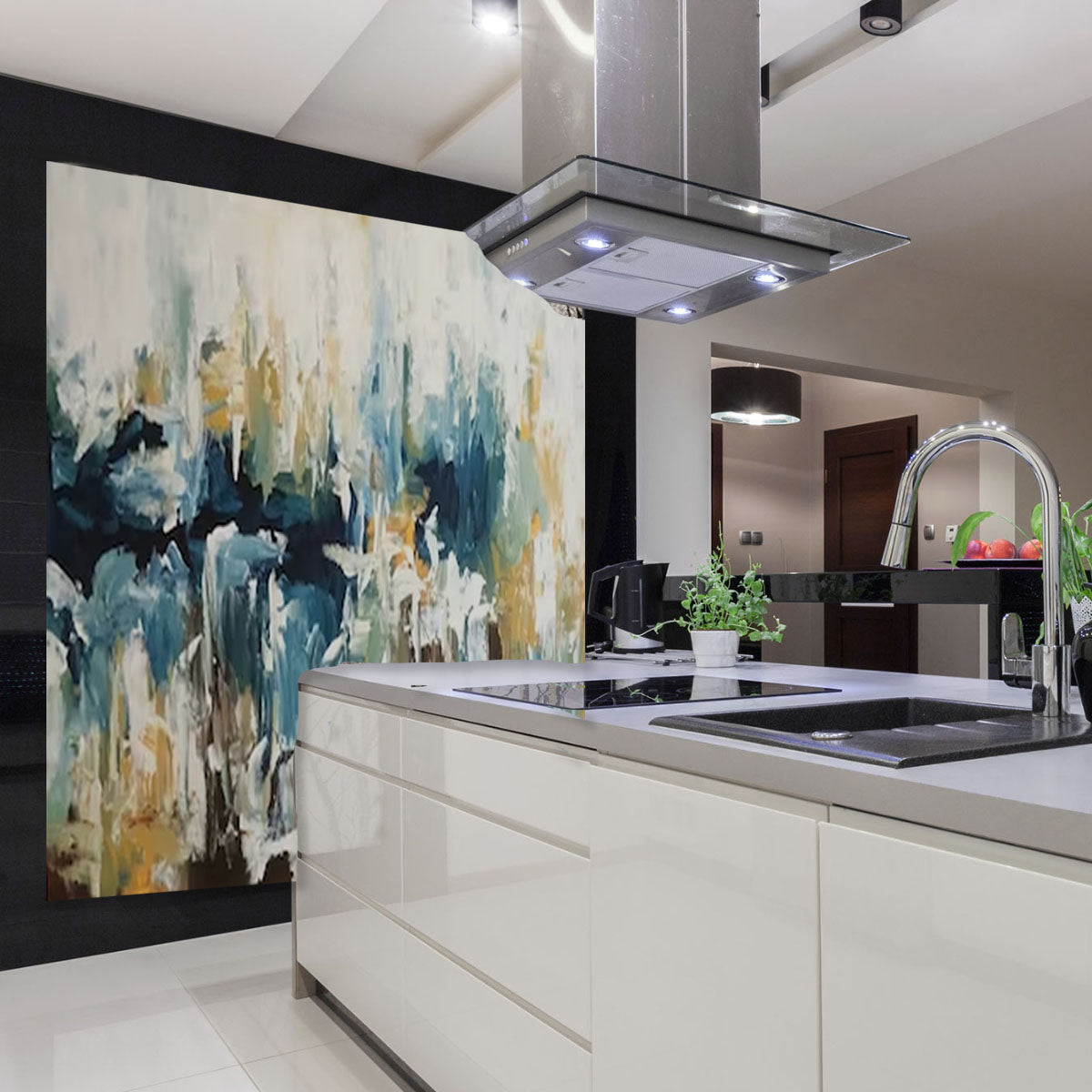The image features a very modern kitchen with a sleek and clean design. The prominent element is a flat-top countertop stove without an oven, positioned next to a stainless steel sink embedded in a grayish-colored countertop. Below the countertop, there are handleless white cabinets and drawers that have a glossy finish. Above the stove area is a stylish ventilation hood with lights, extending up to the ceiling. 

A large piece of abstract artwork dominates the black wall adjacent to the countertop. This painting is vibrant with a mixture of blue, white, yellow, orange, and brown hues, giving a contemporary feel to the space. On the countertop, there is a white pot holding a green plant and what appears to be a coffee pot or a kettle for boiling water. Additional kitchen elements include a black lacquer shelf positioned above the sink, with a plate of apples on it.

The kitchen floor is tiled with white squares, adding to the bright and modern aesthetic. Towards the right side of the image, there's an area with another plant that is partially visible, as well as a door with a light fixture above it. The overall ambiance of the kitchen is one of streamlined modernity and minimalist elegance.